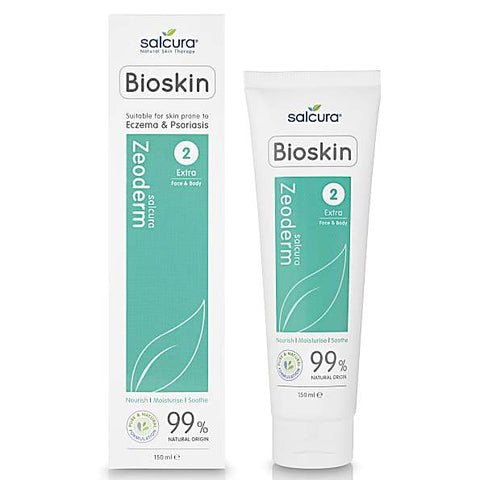The image features a product called "Bioskin Zeoderm" by Salcura. The setup includes the product's white tube on the right and its corresponding box on the left. Both the box and the tube display the company logo "Salcura" at the top, followed by the product line name "Bioskin" in black letters. The packaging prominently notes "Eczema and Psoriasis" under the product name. A green band across both the tube and the box highlights a circled number "2" in white, indicating the product type or step in a regimen. Below this, the product's name "Zeoderm" is displayed. The design also features an outline of a leaf in white towards the bottom, emphasizing its natural qualities. Additionally, both the box and the tube claim "99% natural origin," indicating the purity and natural components of the product. The tube contains a cream designed to nourish and soothe the skin, although the specific ingredients are not detailed in the provided description.